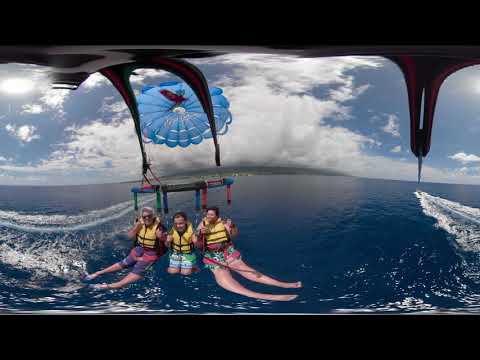In this photograph, taken from the back of a boat, three individuals are preparing to parasail. They are seated at the edge of the boat with their legs and feet submerged in the calm, blue water. All three are strapped into their harnesses and are wearing yellow life jackets. The person on the left is wearing sunglasses and has their legs extended straight, while the person in the middle has their legs pulled up against their body, and the person on the right also has their legs mostly straight but slightly bent towards the center. The blue parasail is already aloft in the sky, tethered to the boat, which has a cover. The serene water glistens with the reflection of the sun, which peeks through the large, puffy clouds in the mostly cloudy blue sky. In the distance, a landmass, possibly an island, is visible on the horizon, adding depth to the peaceful yet exhilarating scene.